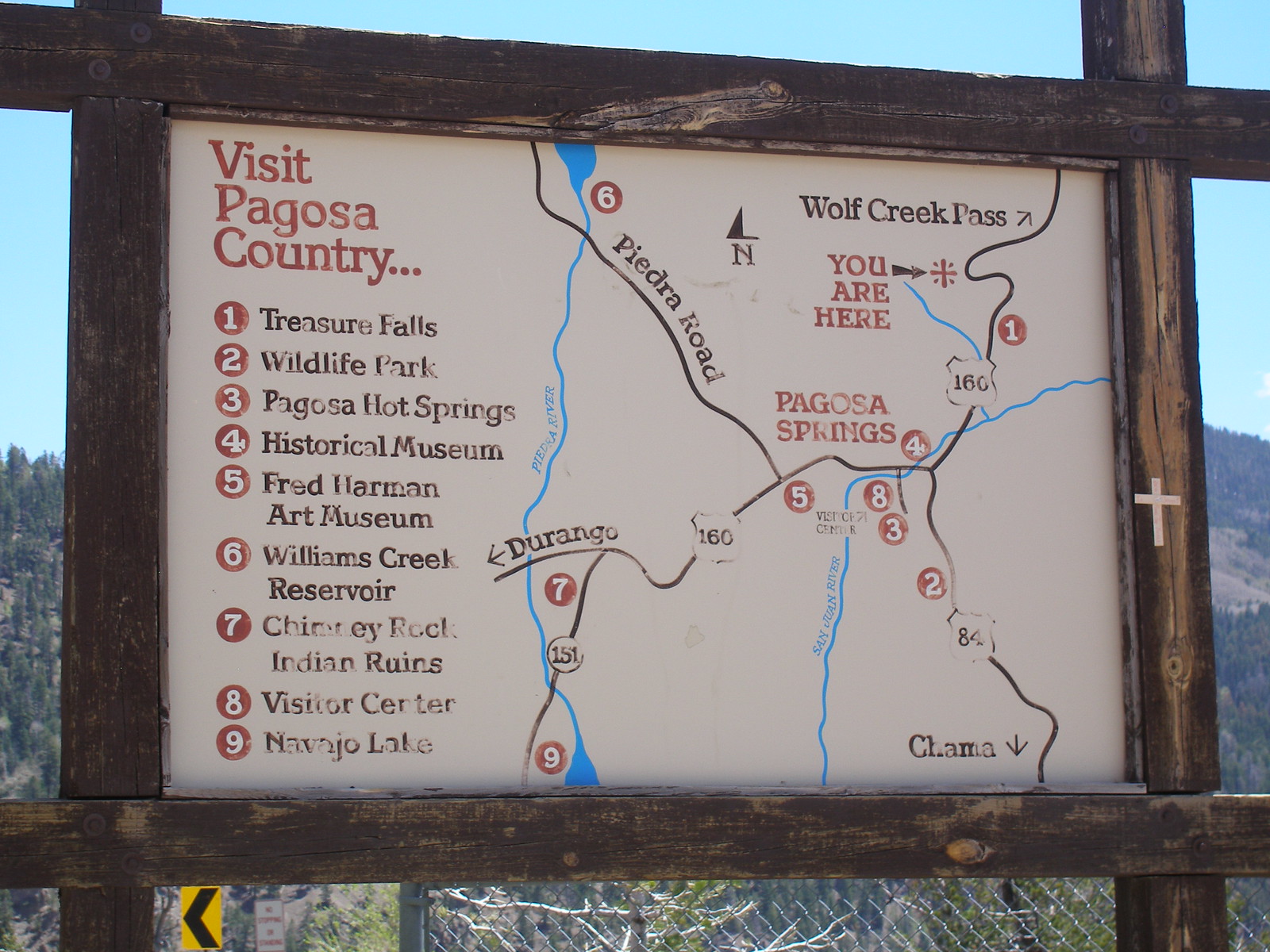The image showcases a detailed hiking map prominently displayed on a large wooden board, positioned centrally in the frame. The map features a tan background accented with colors such as brown, blue, and black. It lists attractions in Pagosa Country, including Treasure Falls, Wildlife Park, Pagosa Hot Springs, Historical Museum, Fred Harman Art Museum, Williams Creek Reservoir, Chimney Rock Indian Ruins, the Visitors Center, and Navajo Lake. The top half of the background reveals a light blue sky, while the bottom half shows a mesh metal fence to the right, and street signs to the left. Beyond the map setup, a tree-covered hillside stretches into the distance with dark green foliage. The entire scene is set against a backdrop of natural beauty, with hints of a rural road nearby, signifying the start of an adventurous journey.